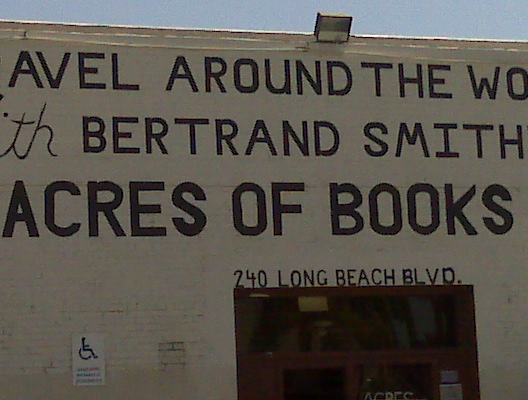The photograph captures the side of a commercial building, possibly a storefront. The building, constructed from light tan stone or brick, appears to be between one to three stories high. The structure features a notable red door frame with sliding doors beneath black text painted directly onto the wall. Some of the visible text includes "Aval," "Around the World," "Bertrand Smith," followed by "Acres of Books" towards the bottom. Above the door frame, the address "240 Long Beach Boulevard" is clearly displayed. Near the left side of the image, a handicap sign is visible, and a square light fixture is mounted above the entrance, presumably to illuminate it. The camera angle points upward from the ground, therefore the very base of the wall isn't visible in the shot.